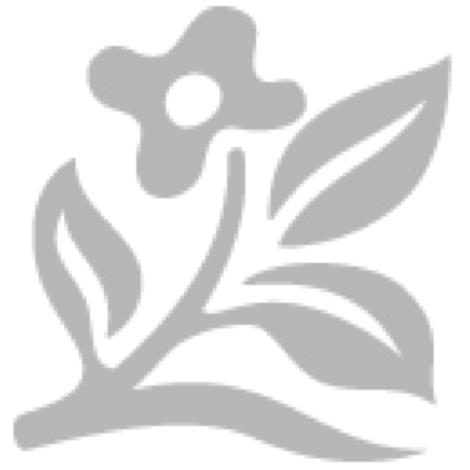The image is a high-quality, professionally edited close-up of dense, overlapping grapevine leaves. Dominating the scene are vibrant red and orange leaves that are more focused and capture immediate attention, especially towards the center. The right side of the image features sections of darker greens and purples, gradually transitioning to yellow and green hues in the middle. On the left, towards the upper part, the coloration shows more green, with the overall composition getting redder and darker towards the edges. In addition to the colorful foliage, the center of the image reveals small, green, nodule-like buds resembling nascent grapes hanging down the vines. The plant's density is highlighted by the fact that no background is visible, making the vivid, layered leaves completely fill the frame.